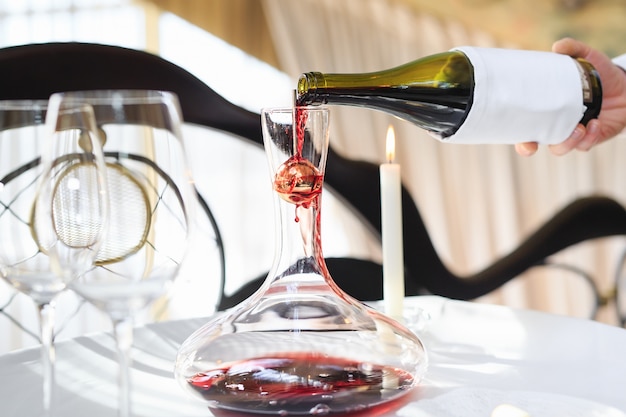The image captures a sophisticated dining scene in what appears to be a fancy restaurant or possibly a wedding setting. Central to the composition is a person’s hand elegantly pouring wine from a green bottle, wrapped in a white napkin, into a unique carafe. The carafe, slender at the top and widening towards the bottom, features a distinctive ball-like mechanism through which the wine is poured. The table beneath this delicate act is draped in pristine white linens and adorned with a lit candle, adding a soft glow to the ambiance. Flanking the carafe are two tall, clean wine glasses, poised and ready for a celebratory toast. In the background, a white cuff on the pouring hand hints at a formal attire, likely a waiter’s uniform. Additionally, the scene includes glimpses of chairs and a black iron railing under the misty blur of natural light streaming in through a window. The unfocused background and gold accents on the table suggest an atmosphere of elegance and class, befitting special occasions like an anniversary or a wedding.